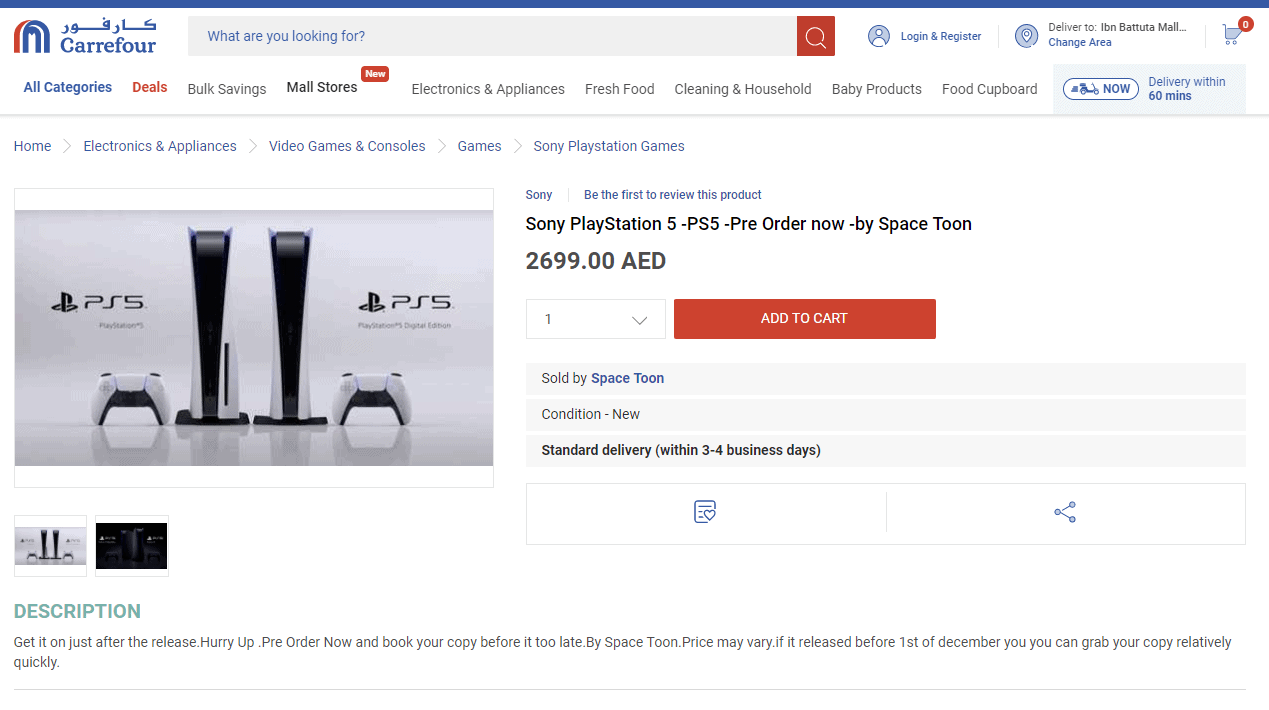The screenshot displays Carrefour’s e-commerce platform. In the top left corner, the page features Arabic-style text indicating the website's branding. Centered prominently is an image of a Sony PlayStation 5 (PS5) console setup. This includes two PS5 towers and two white DualSense controllers. The product description highlights this as a pre-order of the Sony PlayStation 5, offered by Space Tune, priced at 2699 AED.

Beneath the product name, a conspicuous red "Add to Cart" button is visible, signifying that the product can be purchased immediately. Additional details indicate that the item is "Sold by Space Tune," is in new condition, and standard delivery is estimated within three to four business days. In the top right corner, a shopping trolley icon with a red circle and the number "0" denotes that no items have been added to the cart at the time the screenshot was taken.